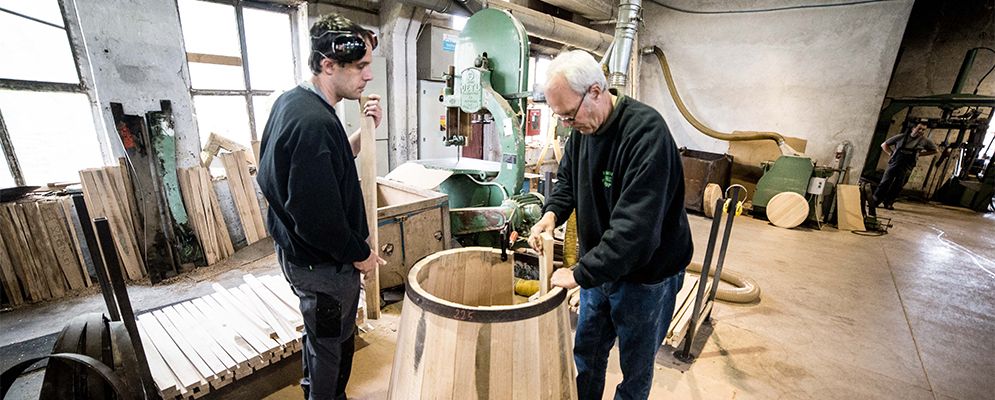In a bustling workshop with tile flooring and white walls, two carpenters are captured in the midst of assembling wooden barrels. The older man on the right, distinguished by his gray hair, glasses, black sweatshirt, and blue jeans, meticulously adjusts a slat into the metal ring atop the partially completed barrel. Beside him, a younger man with brown hair and unused hearing protection resting on his head, also dressed in a black top and jeans, holds another wooden slat. Scattered around them are various nondescript items, including what appear to be pillows and a canvas curtain acting as a wall separator on the right. In the backdrop to the left, rows of neatly stacked wooden slats rest against a palette and wall, ready for use. A machine, likely integral to the barrel-making process, is situated between the two craftsmen. In the background, a third individual watches over the scene, underscoring the industrious atmosphere of this manufacturing plant.